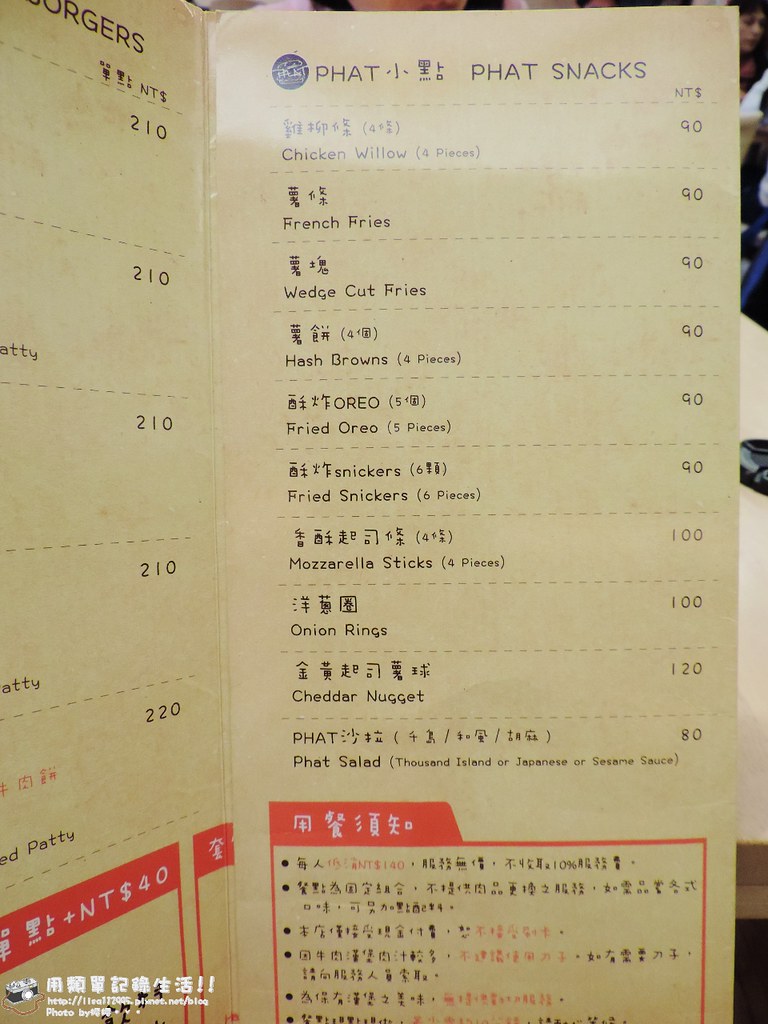This image depicts a single-page menu from a restaurant. The menu is positioned vertically on a light brown table, with part of the table visible to the right side and a strip crossing the top of the picture. The table also features an indistinct blackish-grey item. In the upper right corner of the background, there's a partial view of a woman's face, suggesting she may be another patron of the restaurant. 

In the bottom left area of the image, white symbols are arranged in a row, followed by words and a small icon next to them. The menu itself appears to be made of a sturdier material, thicker than paper but not heavily bound. The design suggests it opens once to reveal the listed items.

The menu focuses primarily on burgers, displaying a series of prices that read 210, 210, 210, 210, and 220. The term "PHAT Snacks" is prominently featured, with "PHAT" creatively spelled with a "P" and "H". It lists the items with their respective icons and prices. There is also a small section highlighted in orange, while another section on the first visible page is outlined in red.